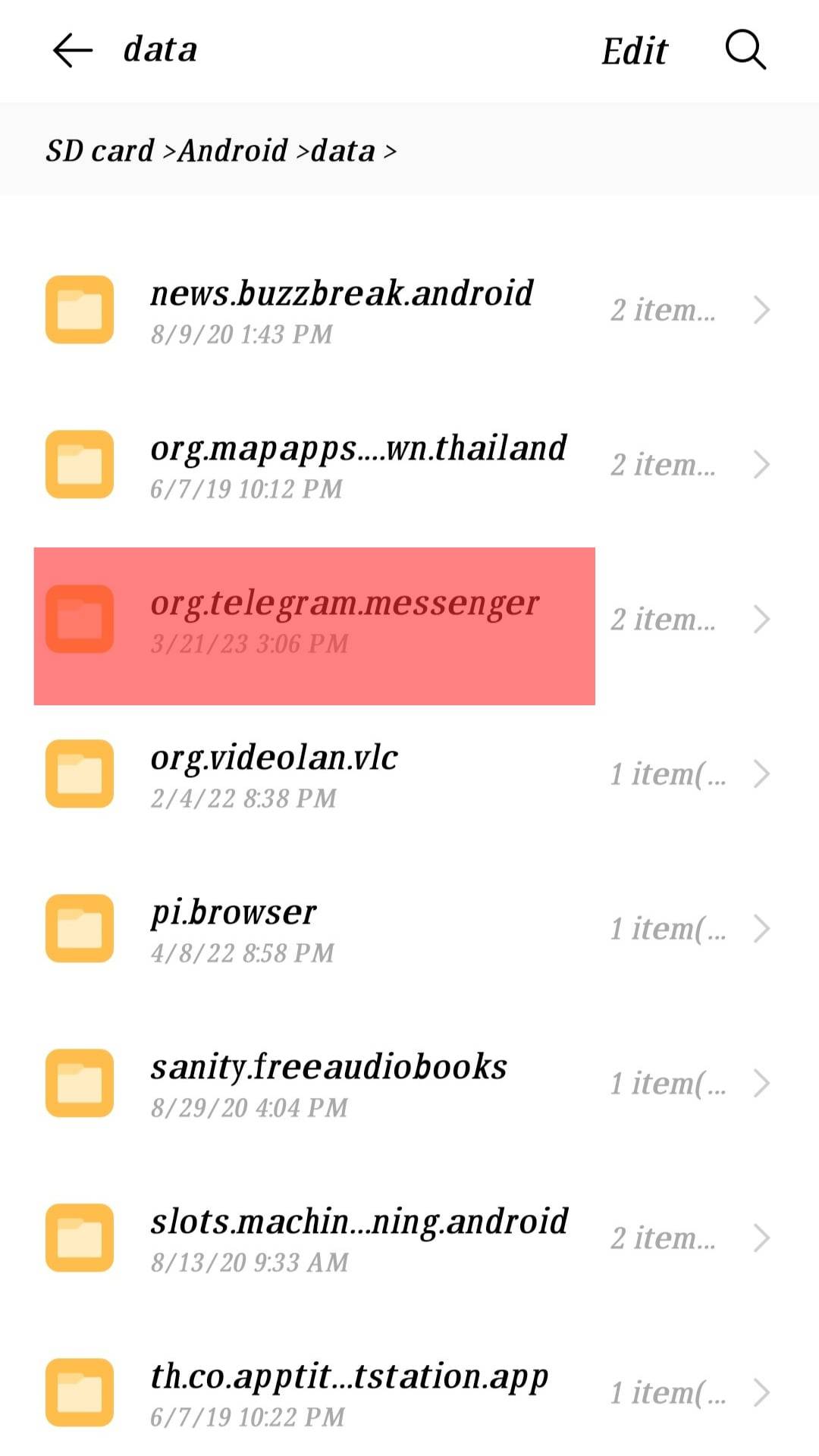This image displays a user interface on a white background with black text. At the top left, there is the word "Data" accompanied by an arrow pointing to the left. On the right-hand side, the word "Edit" is displayed along with a magnifying glass icon. Below these headers, the text reads "SD card, android, data."

The main section features a list of files, each represented by a file folder icon on the left, followed by the name and details of each file on the right. The details for each file include the date and time of the last modification and the number of items within the folder.

1. **news.buzzbreak.android**: Modified on 8/9/20 at 1:43 PM, containing 2 items.
2. **org.mapapps.dot.wn.thailand**: Modified on 6/7/19 at 10:12 PM, containing 2 items.
3. **org.telegram.messenger** (highlighted in red): Modified on 3/21/23 at 3:06 PM, containing 2 items.
4. **org.videolan.vlc**: Modified on 2/4/22 at 8:38 PM, containing 1 item.
5. **pi.browser**: Modified on 4/8/22 at 8:58 PM, containing 1 item.
6. **sanity.freeaudiobooks**: Modified on 8/29/20 at 4:04 PM, containing 1 item.
7. **slots.machine.android**: Modified on 8/13/20 at 9:33 AM, containing 2 items.
8. **th.co.apptit.dot.tstation.app**: Modified on 6/7/19 at 10:22 PM, containing 1 item.

The highlighted entry "org.telegram.messenger" indicates it has particular significance or has been selected by the user. This organized display allows for easy navigation and management of the data files stored within the SD card on an Android device.